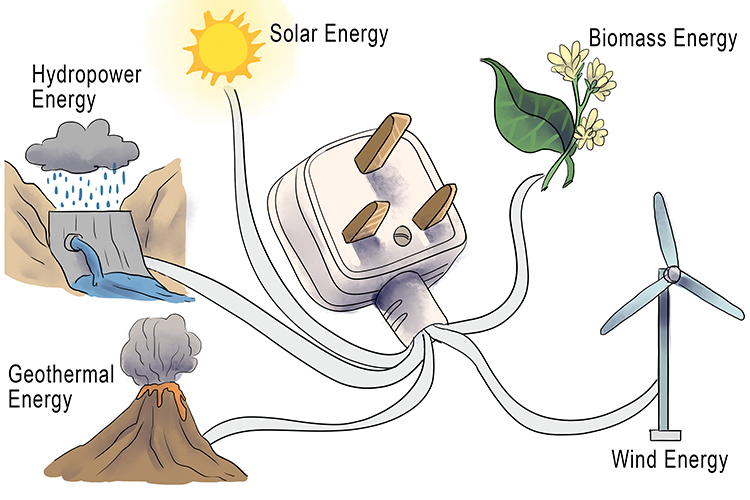The image is a detailed, watercolor-style illustration explaining various energy sources and how they collectively power household devices. On the upper left, labeled "Hydropower," is a rain cloud pouring water into a dam, emphasizing the role of water in energy production. Directly below, on the bottom left, is "Geothermal Energy," depicted by an erupting volcano. Moving to the top middle-left, the sun represents "Solar Energy," highlighting solar power. The upper right features a small flower and leaf, indicating "Biomass Energy." Finally, on the bottom right, a wind turbine stands for "Wind Energy." Each energy source is connected by lines or wires converging to a central point—an electrical plug typical of European outlets. This plug symbolizes how these diverse types of energy can collectively power household devices.